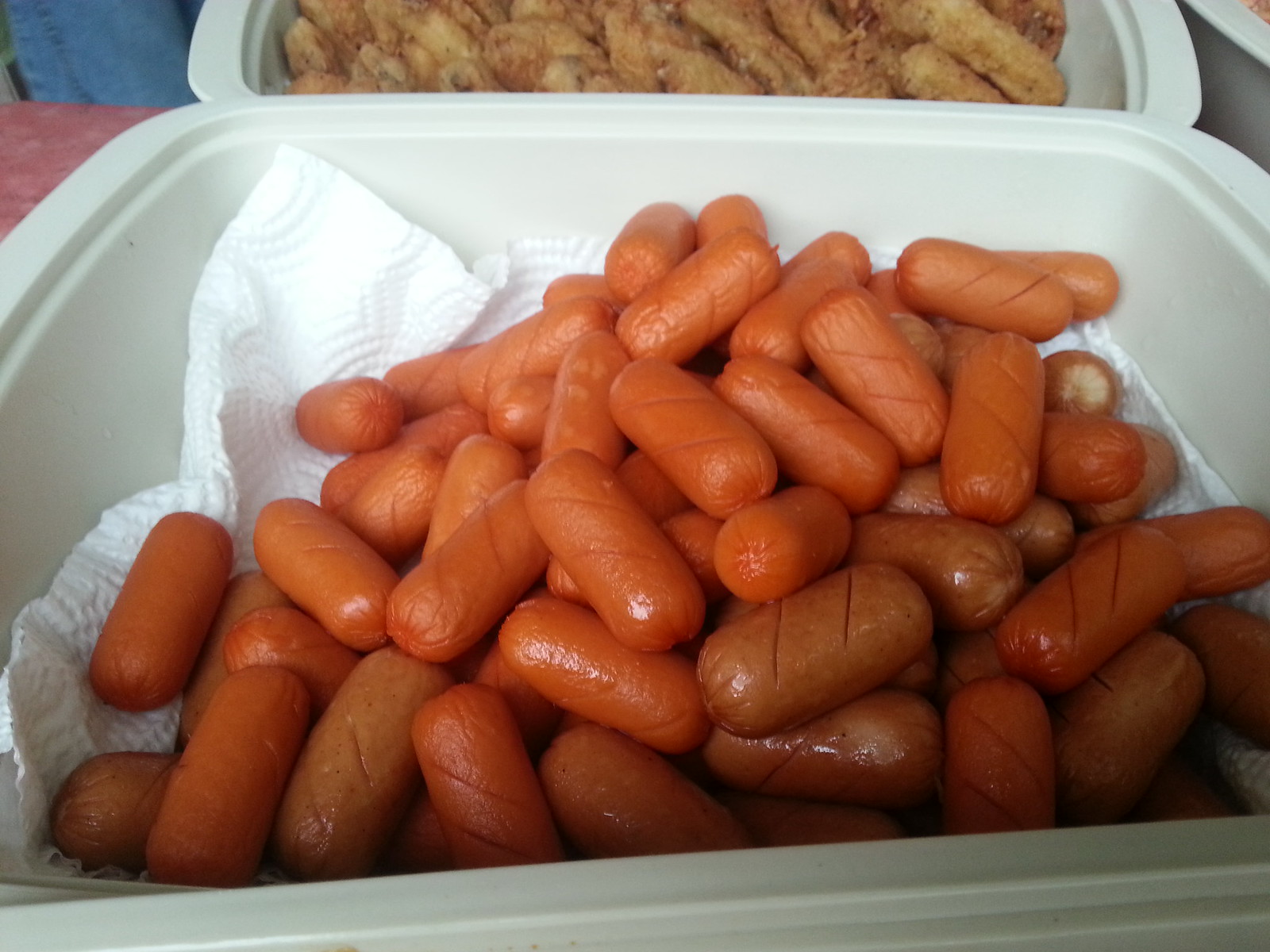This photograph captures a close-up view of two white plastic takeout containers with a variety of food items. In the foreground, a bowl-shaped container lined with a paper towel is filled with numerous mini sausages. These sausages are about the size of a small adult thumb, scored with diagonal lines, and vary in color from a rich, darker brown to a reddish-brown. It's estimated that there are between 50 to 100 of these mini sausages. Behind this, a second container, partially clipped off at the top, holds a pile of golden brown, breaded chicken wings. The chicken wings do not appear cooked hot, suggesting they may have been defrosted from a freezer. This scene is set on a pink-colored countertop with a hint of blue fabric, possibly denim, in the top left corner.